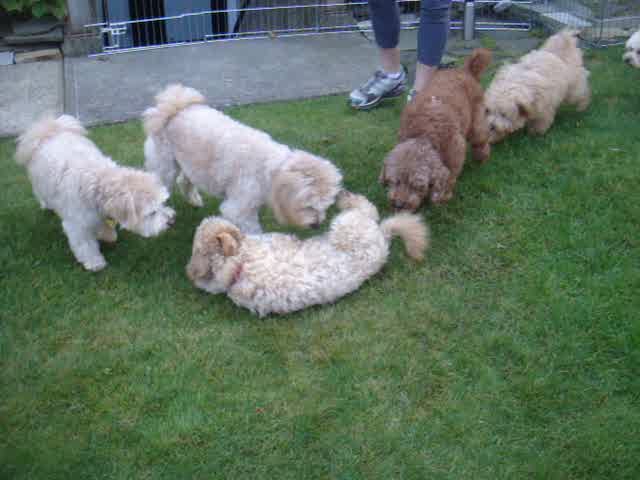This image is a color photograph taken outdoors, likely in someone's backyard or a kennel area. It features five small, fluffy dogs that appear to be a Maltese or Maltese poodle breed. Four of the dogs are cream-colored, while one is chocolate brown. A sixth dog is partially visible, with only its head peeking in from the upper right corner. The dogs are all playing or interacting on a grassy area, with one dog lying down wearing a red collar. The background includes a metal fence and the lower legs of a person, presumably a woman, dressed in blue leggings and sneakers. The dogs have short, curly fur, fluffy ears, and tails. The scene is lively, capturing the dogs in various stages of play and curiosity.